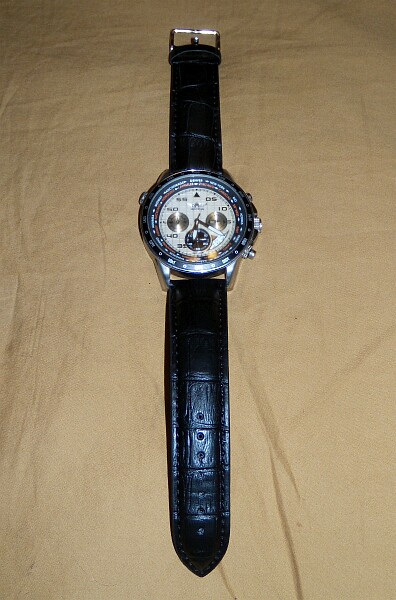In this detailed photograph taken indoors, a watch is prominently displayed in the center against a wrinkled tan fabric background, possibly a bed sheet. The watch features a brown face encased in a silver rim, embellished with various tiny circles and dials, creating a busy and intricate appearance. The background inside the watch face is white, with black numbering and multiple arrows pointing in different directions. There are three silver knobs—one on the left and two on the right side of the watch. The black leather band, which appears to be made from animal skin, is spread open with visible holes on the bottom end and a silver metal buckle at the top. The detailed craftsmanship and contrasting elements of the watch are clearly the focal points of this photograph.